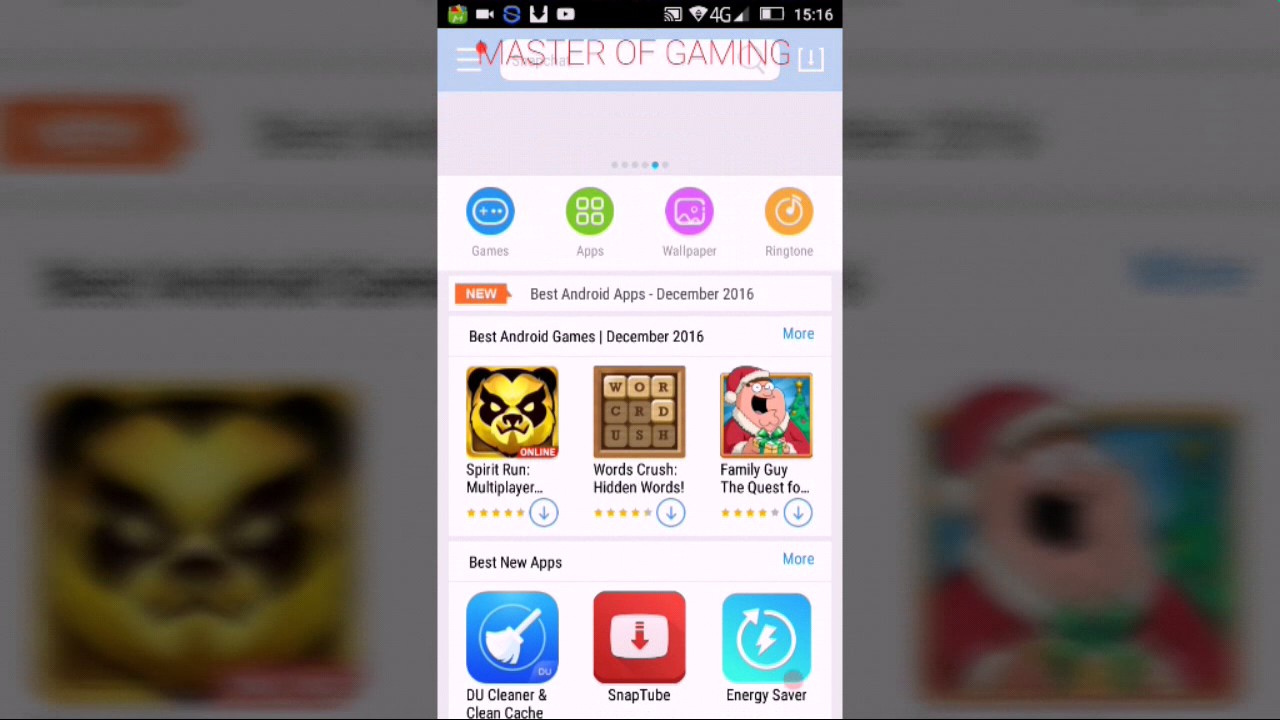A mobile phone screen displays a pop-up, seemingly mirrored by a larger image of the same on a background computer, suggesting the phone's screen is being cast to the computer. The phone screen has a green icon at the top, whose exact function is unclear. Other icons include a video button, a blue 'S', a download button, a YouTube-like 'play now' button, and a 'cast to device' button, reinforcing the idea of screen mirroring. 

The status bar indicates Wi-Fi is connected, 4G network is active, the battery is low, and the time is 15:16. The page viewed on the phone is titled "Master of Gaming." Below this title, there are tabs labeled "Games," "Apps," "Wallpaper," and "Ringtone." The subheading reads, "Best Android Apps December 2016."

The listed apps under "Best New Apps" include:
- **Spirit Run Multiplayer**: Features an image of a golden panda with predominantly black features.
- **Word Crush, Hidden Words**
- **Family Guy, The Quest**
- **DU Cleaner and Clean Cache**

Additionally, "SnapTube" and "Energy Saver" are listed as notable apps.